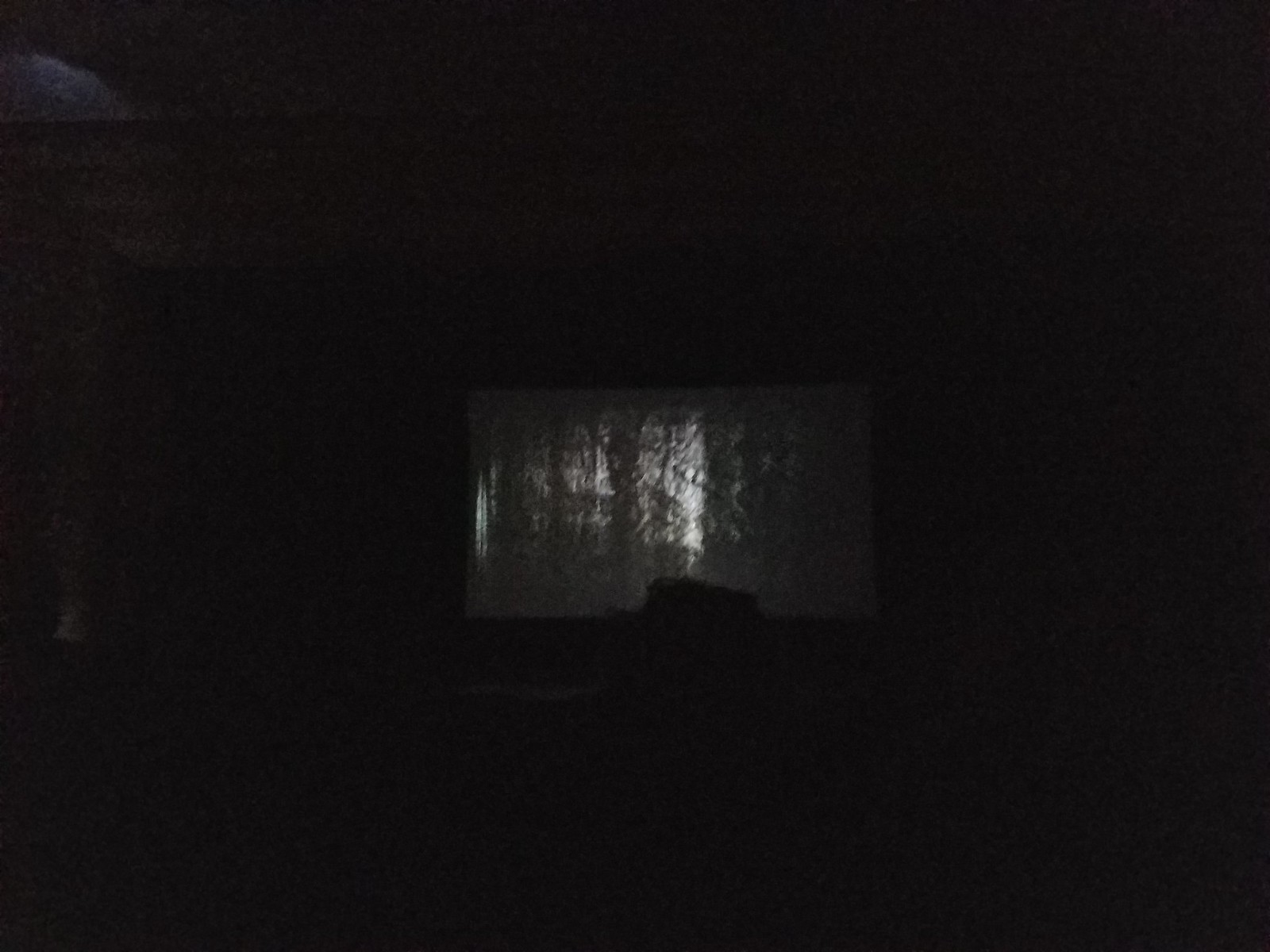This image is a grainy, color photograph with a noticeable, ambient rainy effect upon close inspection. Predominantly engulfed in darkness, the center of the image features a horizontally oriented, rectangular shape. This central element is suggestive of a window, covered by a piece of tautly stretched plastic. The plastic exhibits a silvery hue and captures light reflections emanating from behind the viewer, possibly even reflecting the moonlight, indicating an outdoor setting. The plastic's surface displays distinctive textures, with noticeable bunching or folding in some areas. Surrounding the rectangle, one can discern the faint outline of a frame, potentially indicative of a wooden house frame, particularly visible along the top and the left side of the rectangle.